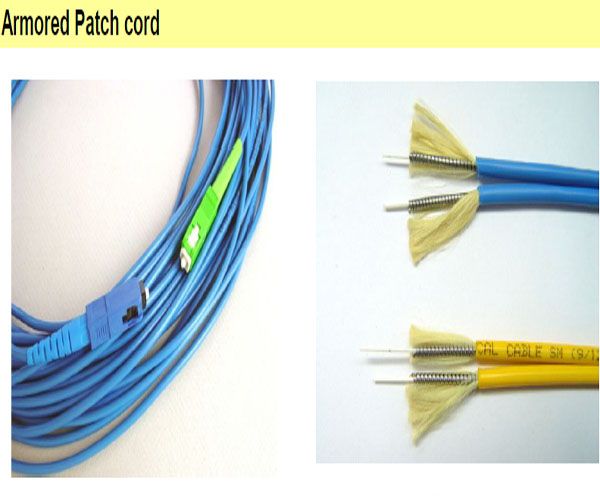The image depicts a detailed view of a coiled wire setup. At the top, there's a molded patch cord in black, prominent against a rectangular yellow section background. On the left side of the image, a half coil of blue plastic wire can be seen, featuring a blue connector at one end and a vibrant neon green connector at the other. Additional details reveal a pair of blue insulated conductors in the upper portion on the right side, each showing a silver rod with spiral springs inside, accompanied by soft, pale yellow threads that resemble yarn. Below it, another pair of insulated conductors appears in yellow, similarly exposing spiral springs and yellow threads. There is a visible marking on the yellow insulated plastic that reads "CAL cable SM, bracket line stroke 12." The overall background on the right side of the image is light blue, providing a clear contrast to the intricate details of the coiled wire and its components.